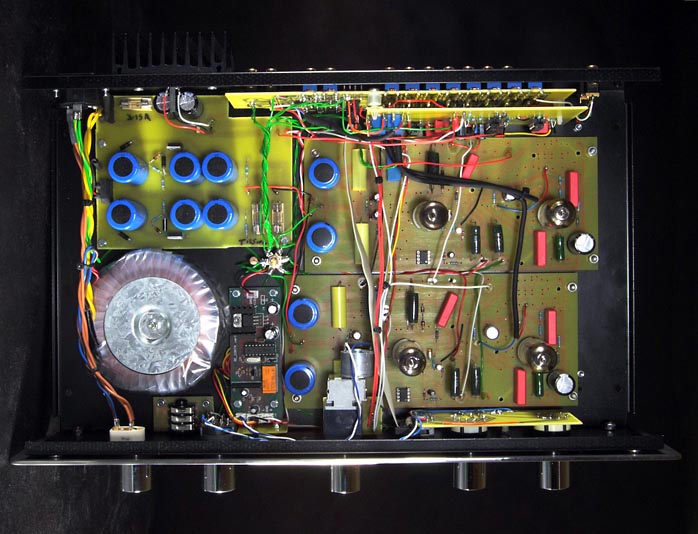This high-quality photograph captures an aerial view of a complex circuit board. The board features several black knobs prominently displayed in the foreground, attached to a black plastic body. A multitude of vibrantly-colored wires, including green, yellow, red, gold, and orange, are meticulously organized and held in place by tiny black clips. The board is also populated with various components such as blue and black cylindrical capacitors, as well as a plastic-covered circle topped with silver. Additionally, silvery, gold, and black square pieces are interspersed among the components. The image showcases numerous black and blue circular objects, as well as additional red and blue wires. Thin red and black objects are also visible, highlighting the intricate and detailed nature of the circuitry.